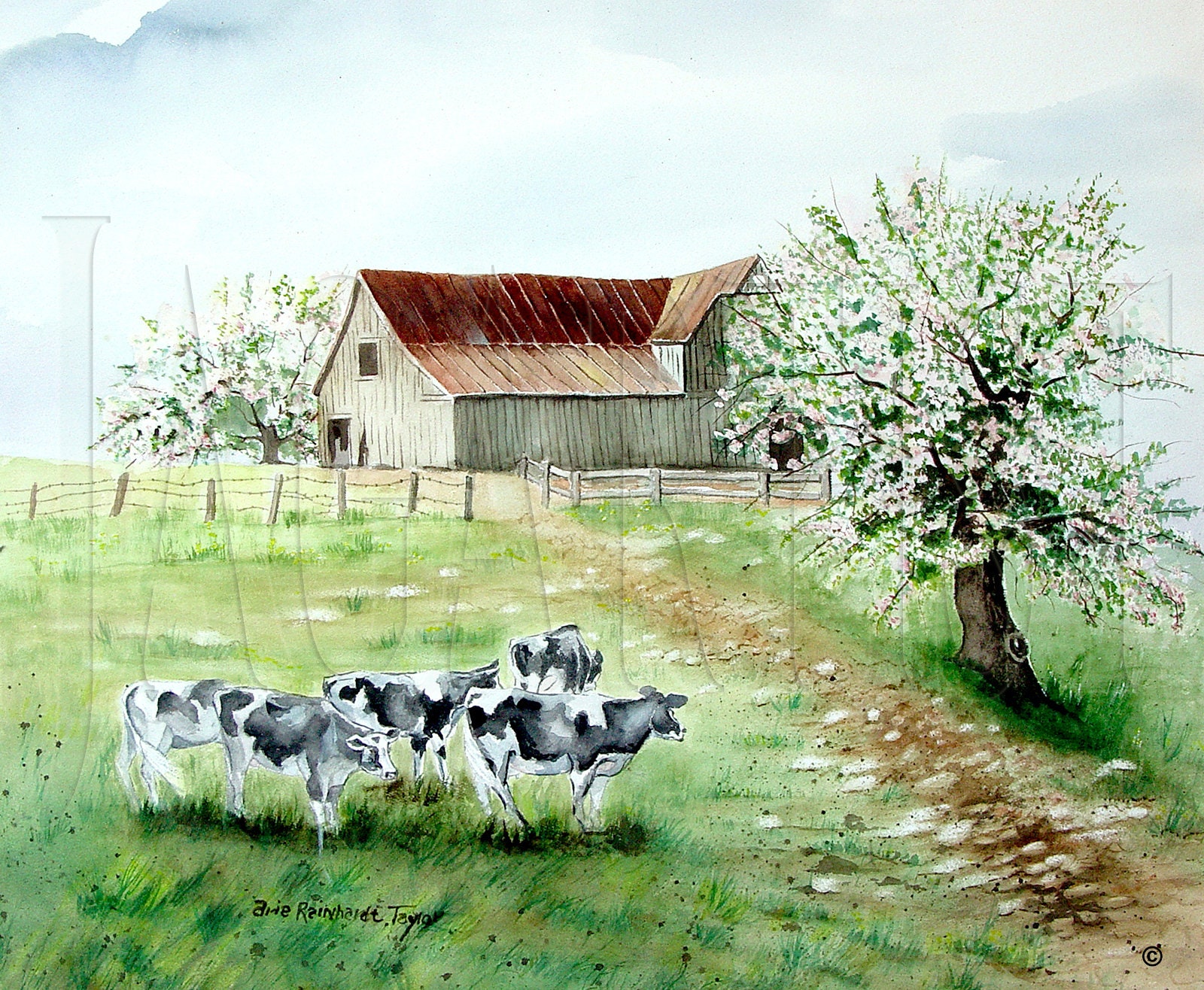This is a detailed watercolor illustration of a pastoral farm scene, with some elements rendered in mixed media. The foreground showcases five black and white Holstein cows standing together in a grassy pasture, all facing toward the right. To the right of the cows, a dirt and stone pathway winds its way from the lower right-hand corner towards the middle of the image, leading to an open gate. The path appears well-trodden, suggesting frequent use.

Flanking this path is a deciduous tree adorned with green leaves and a profusion of white and light pink flowers, creating an eye-catching display. A barbed wire fence marks the boundary of the pasture on the left, while an irregular wooden rail fence appears on the right. The middle ground features a brownish-red roofed barn or farmhouse with weathered gray vertical siding. Beyond the barn, another flowering tree, similar in appearance with white blooms, adds to the pastoral charm of the scene.

The sky above is painted in pale shades of watercolor pastel blue, enhancing the tranquil atmosphere. The bottom right corner of the image bears the name Amy Reinhardt Taylor in small, black handwriting, signifying the artist's signature. The overall composition captures the rustic beauty and serenity of farm life with intricate, harmonious details.